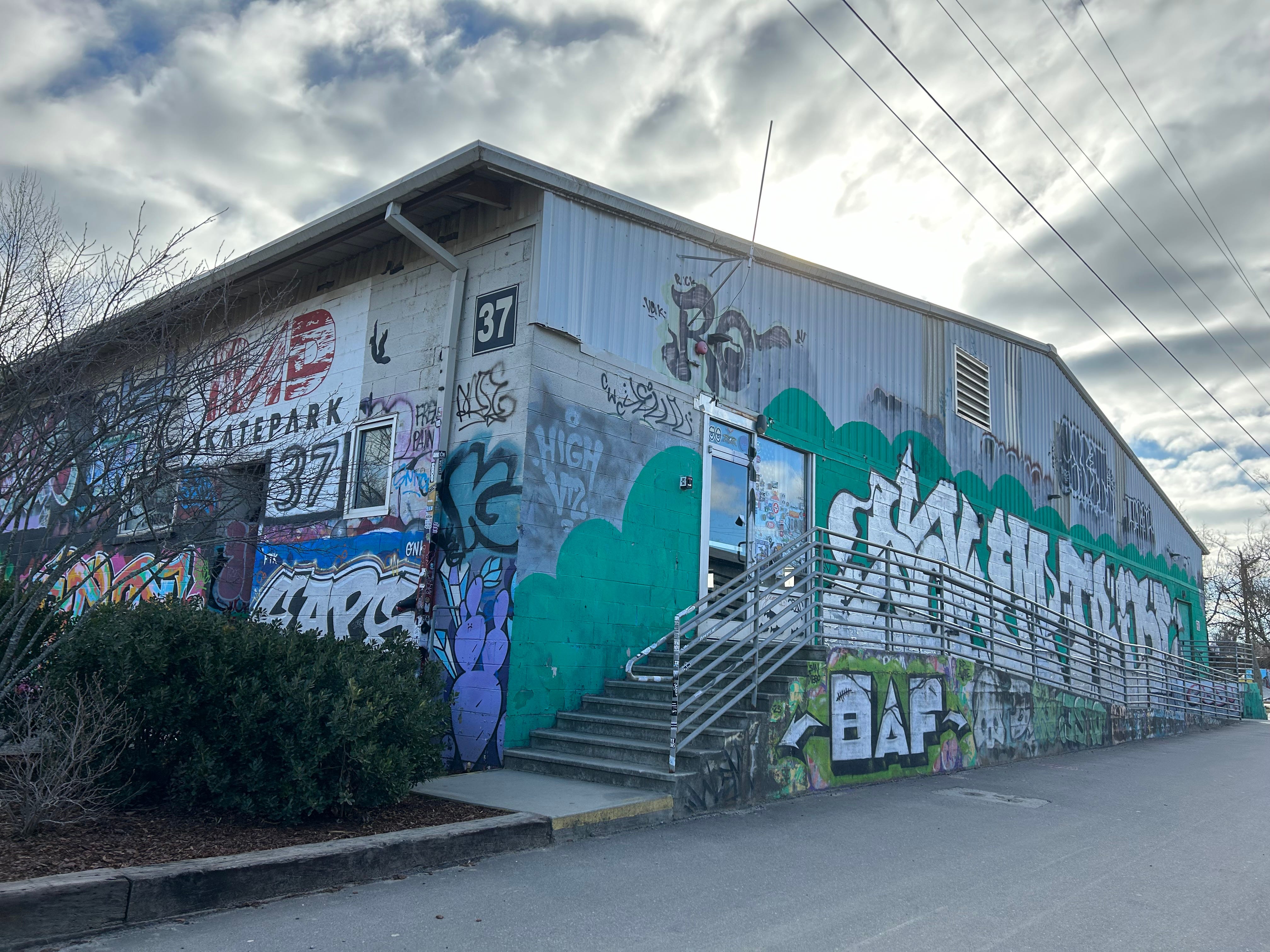This horizontally oriented, realistic photograph captures the exterior of a one-story building, likely a skate park or retail store. The setting is outdoors during the day with a blue sky dotted with clouds allowing sunlight to peek through. The structure resembles a warehouse made of cinder blocks and some corrugated metal, and it is extensively covered in colorful graffiti, primarily in greens, blues, oranges, lighter blues, whites, and pinks. "Skatepark 37" is clearly written in black font on a white section of the building, suggesting it may be the name of the facility. The building also features a glass door accessible via a stairwell, accompanied by a ramp with a railing on the right side. The bottom of the image shows a gray paved area, and a few bushes and power lines are visible in the scene as well.